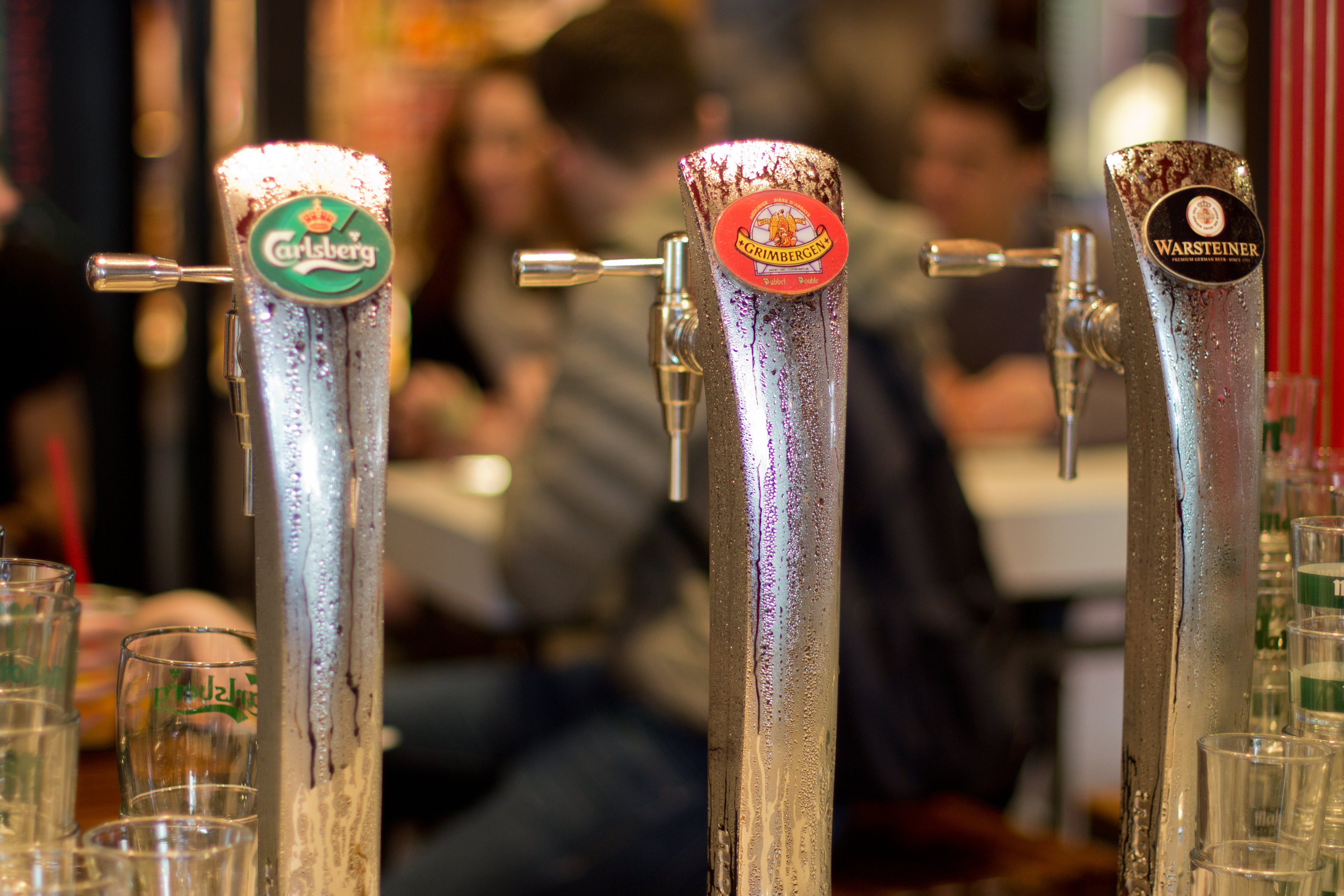The photograph captures a lively bar scene, with the focal point being three silver bar taps, each adorned with condensation and unique branding. On the left, the Carlsberg tap features a circular green logo crowned with gold, inscribed with the brand's name in white. The middle tap showcases a brown-orange Grimbergen logo with a yellow band, distinctly reading "G-R-I-M-B-E-R-G-E-N." The rightmost tap, for Warsteiner, is marked by a black circle and a white logo, highlighted with gold lettering. 

In the bottom left corner, seven clear pint glasses, adorned with green logos, are clustered together, with a patron's arm and a long red straw subtly visible behind them. To the right, six similar glasses are neatly arranged. Beyond the bar taps, the background reveals a slightly out-of-focus white table where three individuals gather. A man, dressed in blue denim jeans, a gray jacket, and a black backpack, sits on the edge of the table facing away, engaging in conversation. Opposite him, a woman with long hair appears to be wearing a black jacket and gray shirt, while to her right, another man with short dark hair dons a black t-shirt. The silver taps, detailed with elegant pink and red highlights, lead the viewer's eye into the rich and bustling atmosphere of the bar.